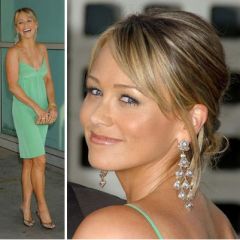This image showcases two professional photographs of a woman, possibly a celebrity, positioned side by side. 

On the left, the full-body shot captures her wearing a dress, looking to the left, and laughing. Her joyful expression and the elegant fall of her dress are highlighted. 

On the right, a close-up image focuses on her from the shoulders up, depicting her glancing back at the camera with a composed and engaging look. 

The image lacks any text, allowing the viewer to focus solely on the subject. Dominant colors throughout the image include shades of green, light green, tan, gray, silver, and brown. Both photographs seem to be taken indoors under professional lighting, enhancing the subject's features and the overall aesthetic. The larger size of the right-side photo draws more immediate attention, creating a balanced yet dynamic composition.